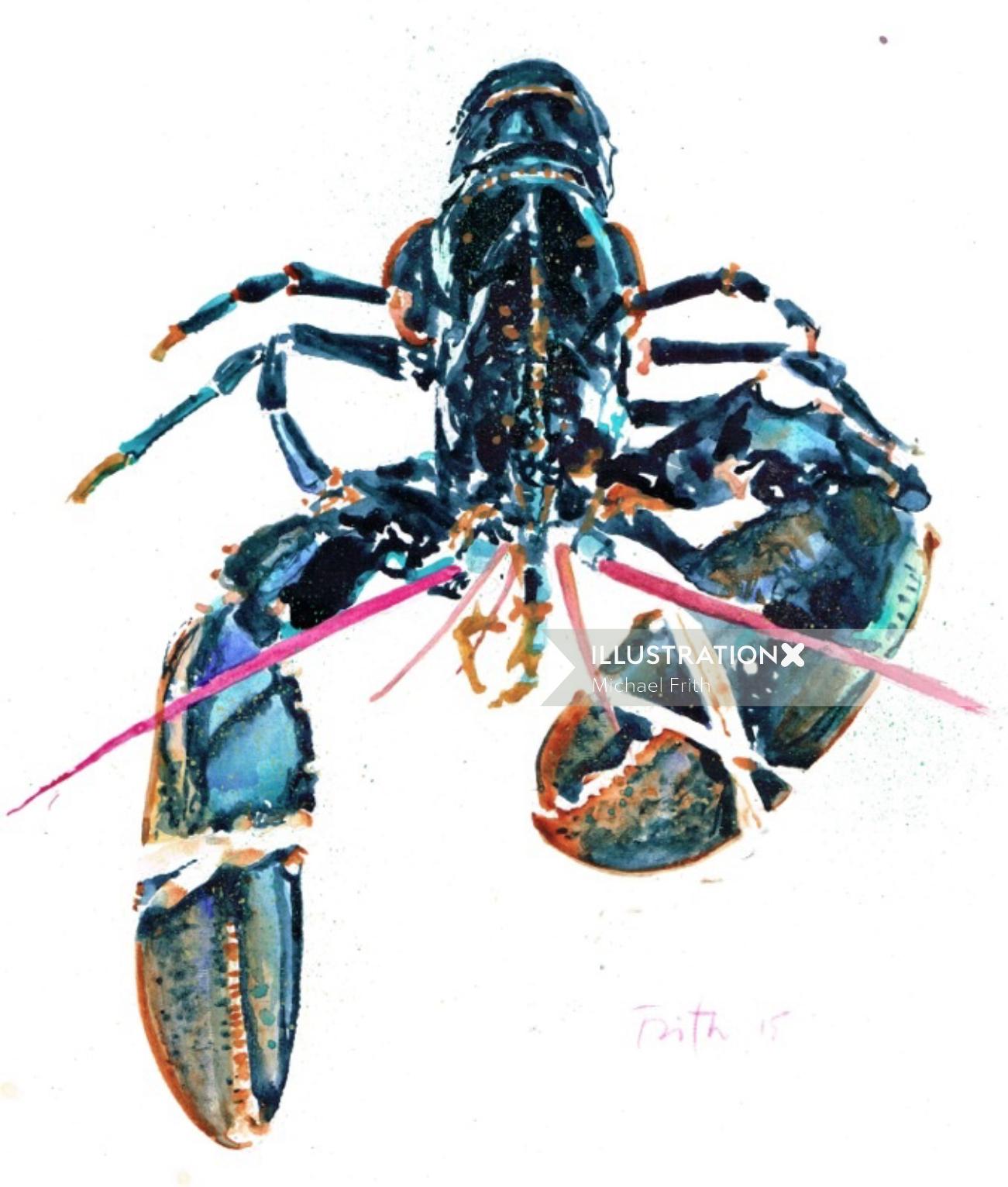The image is a detailed, color illustration of a lobster in a portrait orientation with a predominantly blue and black hue, complemented by pink highlights, especially on the tentacles. The lobster's body is centrally positioned towards the top of the illustration, facing the viewer. It features six segmented legs, three on each side, with the tips shaded in brownish tones. The large claws, depicted with greenish-orange textures and secured with white twist ties, are positioned with one hanging down on the left and the other bent towards the lobster's mouth on the right. The composition has a watercolor style, set against a white background. A watermark in white text at the bottom right corner reads "Illustration, Michael Frith."